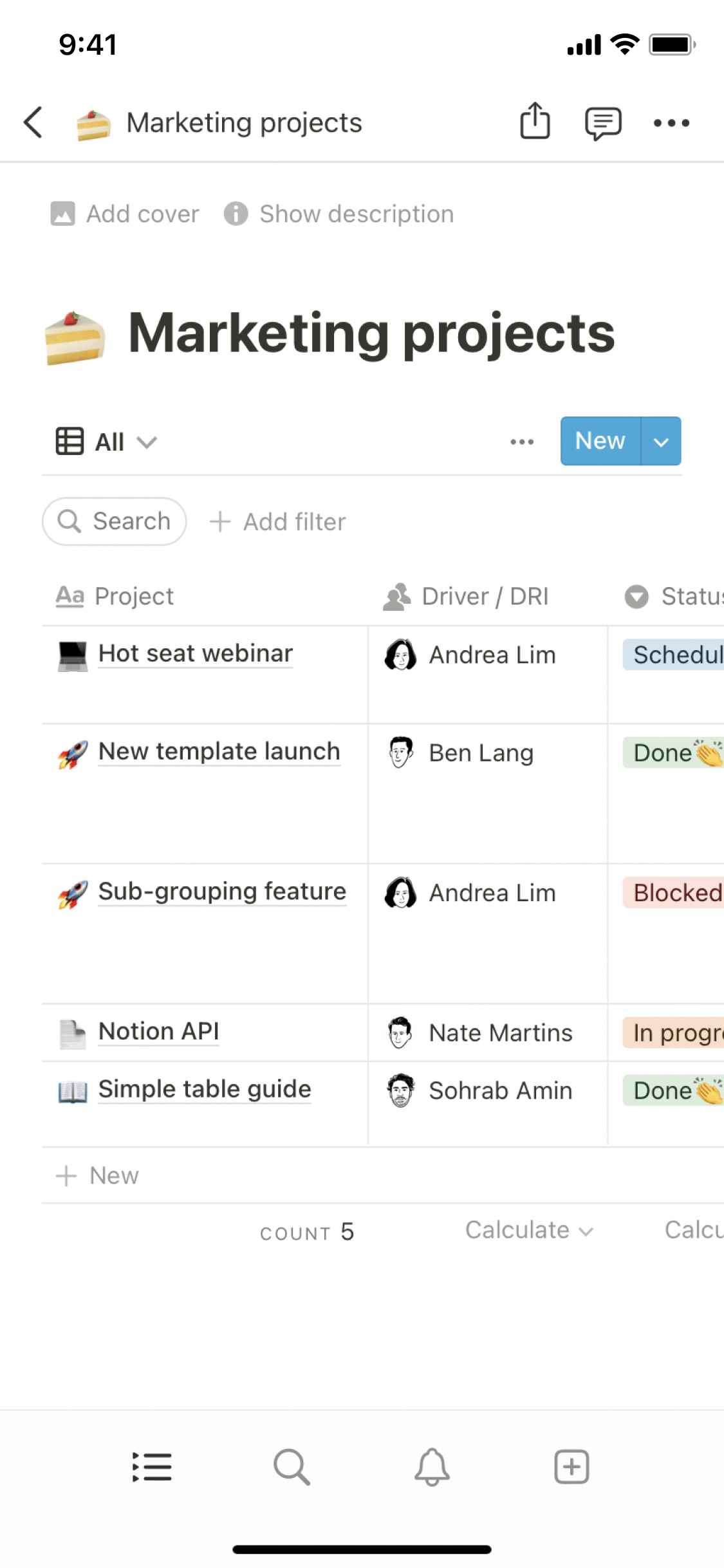A screenshot from a tech company's project management application. The page title reads "Marketing Projects," accompanied by a small icon of a cake with a strawberry on top. The interface has a light mode with a white background. There is a back button for navigation at the top.

The main section displays a table listing five projects: "Hot Seat Webinar," "New Template Launch," "Sub-grouping Feature," "Notion API," and "Simple Table Guide." Each project entry includes additional columns labeled "Driver/DRI" (likely indicating the project lead) and "Status." 

- **Hot Seat Webinar:** Status - Scheduled
- **New Template Launch:** Status - Done
- **Sub-grouping Feature:** Status - Blocked
- **Notion API:** Status - In Progress
- **Simple Table Guide:** Status - Done

Users can click on each project for more detailed information. The bottom of the page shows a project count, displaying "Count: 5."